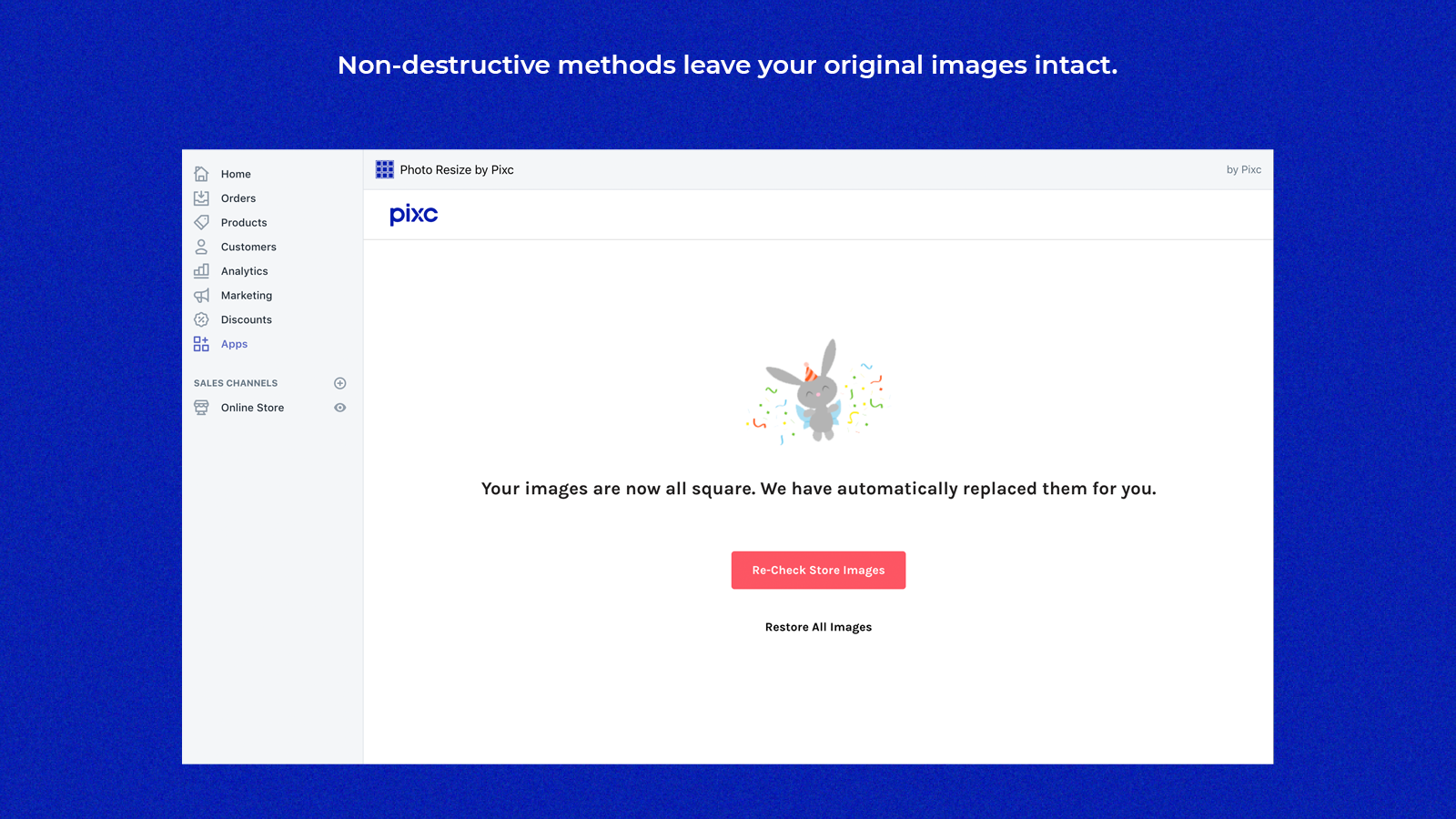Screenshot of a web page with a dark blue background featuring a white font header that reads, "Non-destructive methods leave your original images intact." Below the header, there's a large white rectangular box. At the top of this box, it states, "Photos resized by PIXC," alongside a small blue icon consisting of nine square boxes. Beneath this, the text "PIXC" is displayed in blue.

On the left side of the webpage, there's a vertical navigation menu featuring a list of options: 
- Home
- Orders
- Products
- Customers
- Analytics
- Marketing
- Discounts
- Apps

Each item on the list has a corresponding icon to its left. Below this list is the category title "Sales Channels," followed by the item "Online Store."

The main section of the white rectangular box occupies most of the area, characterized by its white background. At the center, there's a small gray bunny with blue wings, wearing a party hat, surrounded by confetti. Beneath this illustration, the text reads, "Your images are now all square. We have automatically replaced them for you."

At the bottom of this message, there's a red rectangular button labeled "Recheck Store Images," and below it, another option, "Restore All Images."